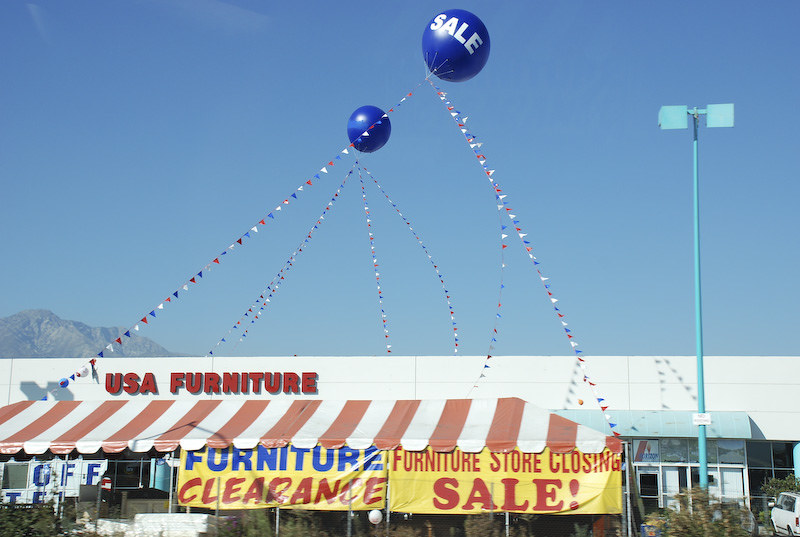The photograph captures a bright, clear blue sky with minimal clouds, save for a slender line of clouds in the upper left corner. In the backdrop, a range of greyish-white mountains can be seen on the bottom left corner, underscoring the natural beauty of the scene. Dominating the foreground is a large, long building identified as a furniture store named "USA Furniture," which is prominently displayed in bold red letters across its predominantly white facade. The storefront is accentuated by a red and white striped awning, serving as a partial covering above the entrance. Below the store's name, a yellow banner inscribed with "Furniture" in blue and "Clearance" in red announces ongoing promotions, alongside another yellow sign that warns of a "Furniture Store Closing Sale" in striking red letters. The scene is further animated by bright blue, reflective balloons emblazoned with the word "SALE" in white letters, hovering above courtesy of long strings adorned with red, white, and blue flags. A solitary white car and a few small bushes are visible near the store's entrance, where various items appear to be piled up under the awning. The image harmoniously blends natural elements with vivid, promotional details of the bustling furniture store.